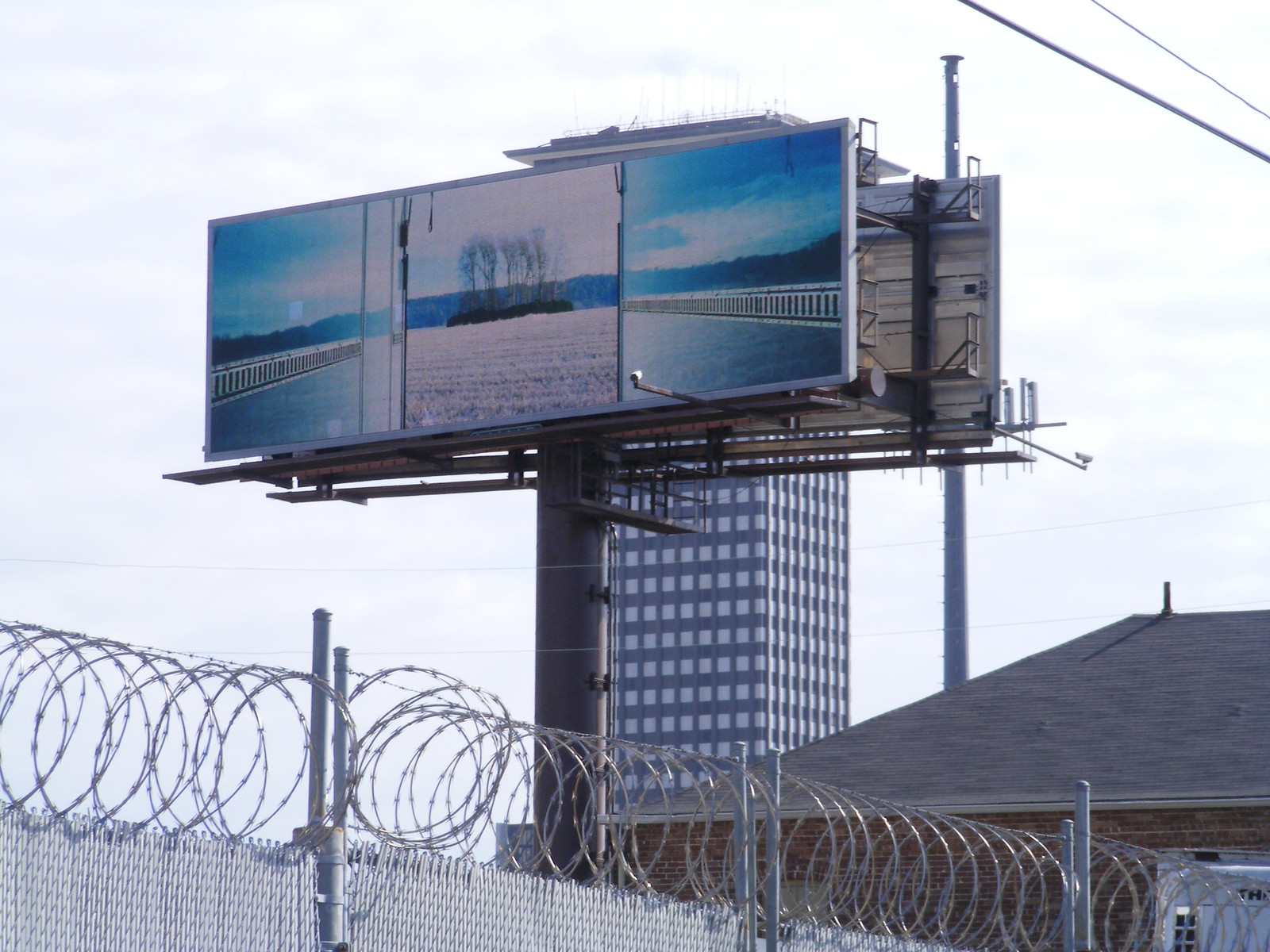Captured from a first-person POV, this image highlights a billboard standing behind a chain-link fence topped with barbed wire. The fence is supported by evenly spaced poles. The billboard itself is mounted on a single, black cylindrical pole and features a display on its front and back. In this scene, we are viewing the front of the billboard from a slight distance, likely taken from a sidewalk towards its right-hand corner. 

The billboard's display showcases a dual image of a walkway or road, flanked by railings on both the left and right sides. Centrally, the image reveals a lush field or sea bordered by green bushes and tall, leafless trees in the background. Below the billboard, partially obscured, stands a brick house with a triangular-shaped roof. Farther in the background, a towering skyscraper stretches towards the cloudy sky, adding an urban layer to the serene landscape depicted on the billboard.